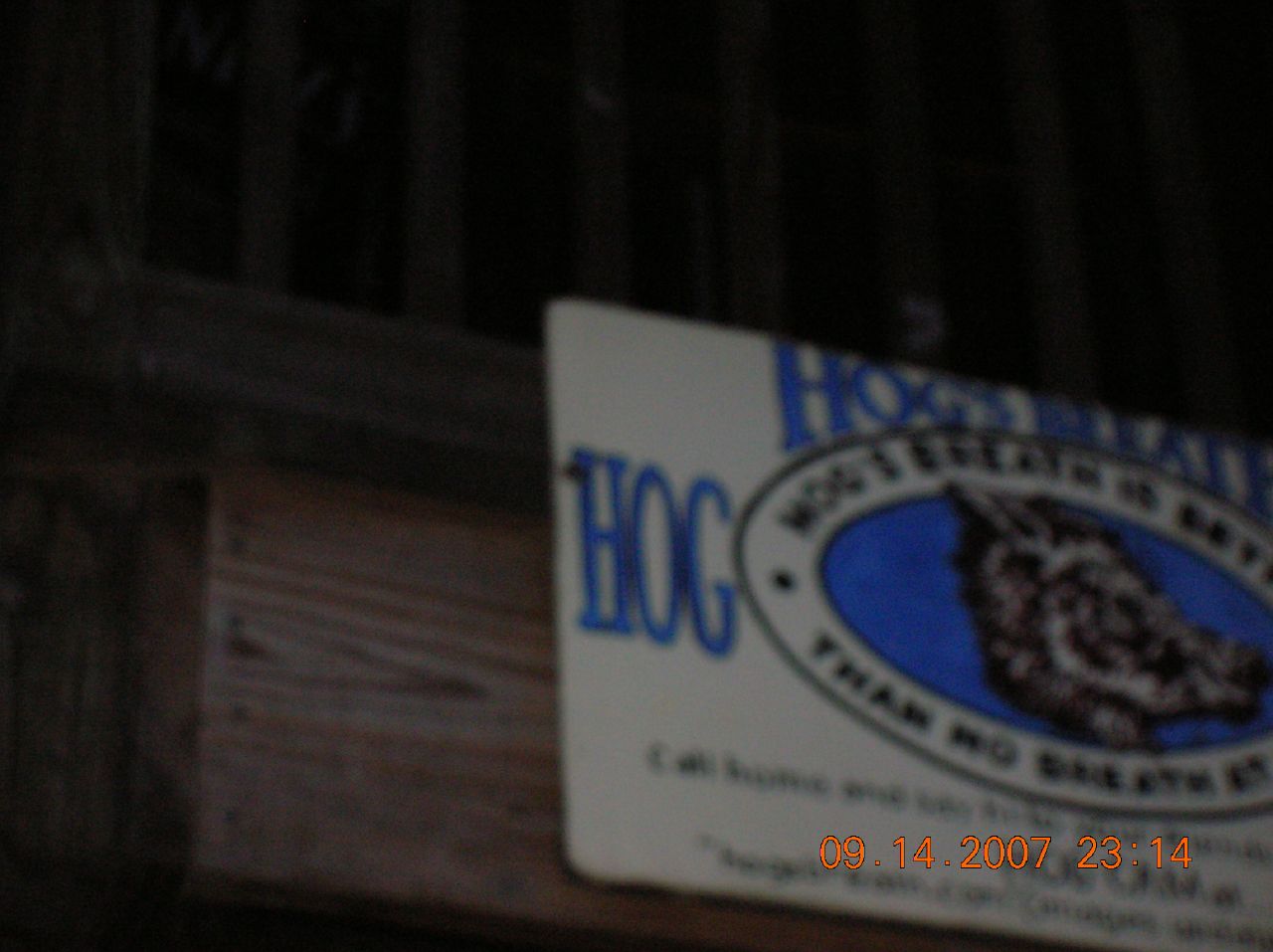In the bottom right corner, the image displays a timestamp reading "09.14.2007 23:14." The background features a wooden wall with windows situated at the top left and top center. In the foreground, a sign prominently reads "Hog's Head" encased within a white circle bordered in black. Inside this circle, the word "Hog" is written in large, bold, blue letters, above a filled-in blue circle depicting the side profile of a hog’s head. The text at the bottom of the sign is challenging to decipher due to its blurriness and low resolution, which imparts a grainy texture to the overall image.